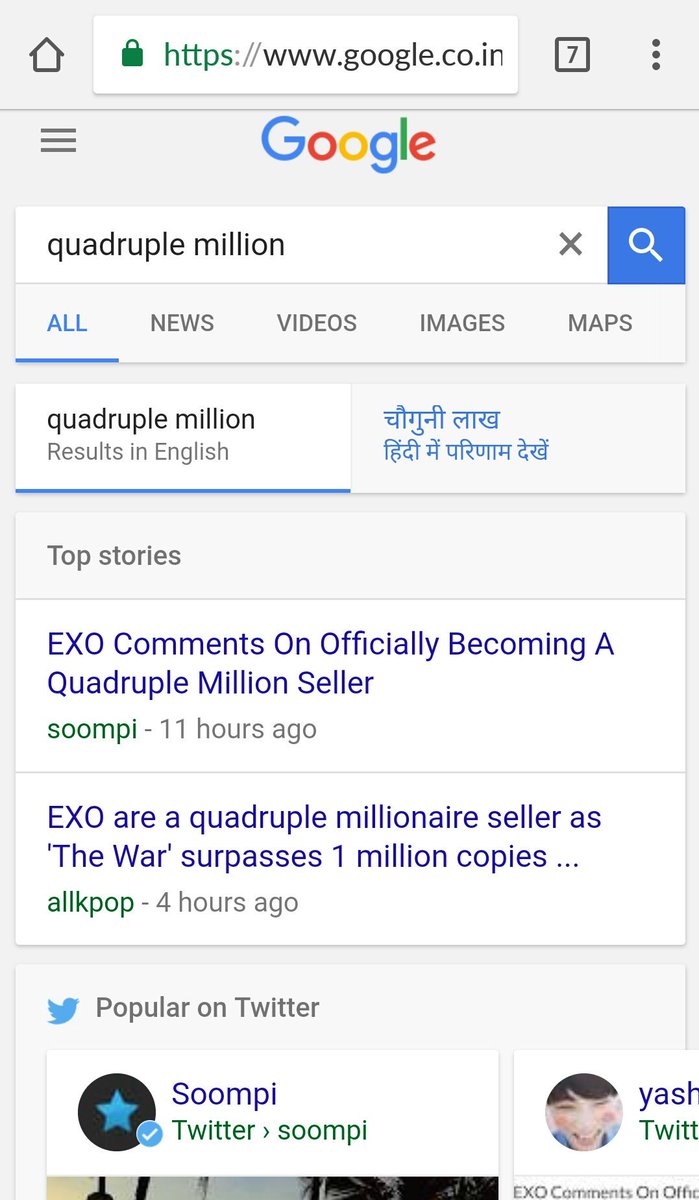The image depicts a Google search results page on a mobile device. The URL displayed in the search bar is www.google.co.in, suggesting an Indian regional domain. The iconic, colorful Google logo is visible underneath the search bar, where the query "quadruple million" has been entered. A blue search button with a magnifying glass icon is positioned next to the search bar. Below this, a navigation menu with options for "All," "News," "Videos," "Images," and "Maps" is underlined in blue, indicating active links.

The search results indicate "quadruple million results" in a box with English and possible Arabic writing in a gray box beneath. The top result, labeled "Top stories," features an article with the headline "EXO comments on officially becoming a quadruple million seller" from Soompi, marked in green and dated 11 hours ago. Another result reads "EXO are a quadruple millionaire seller as the war surpasses one million copies" listed from AllKPop in green, 4 hours ago.

Additionally, there's a "Popular on Twitter" section with partially visible content such as "Soompi" and another cut-off Twitter handle "Yash something," followed by more truncated information at the bottom of the image.